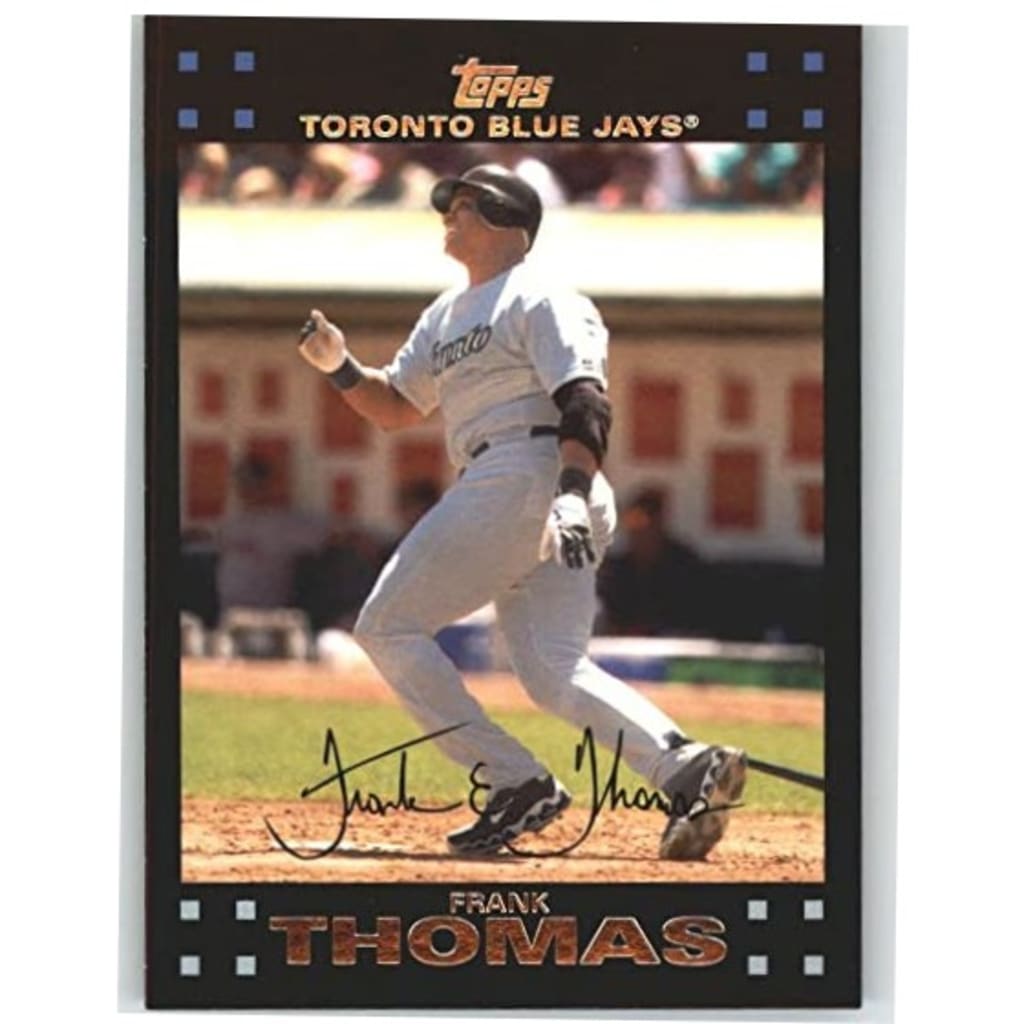This image features a Topps baseball card of Frank Thomas from the Toronto Blue Jays. The card is vertically rectangular with a black frame and a distinctive design featuring four spaced-out blue squares in each of the top corners and light gray squares in each of the bottom corners. Positioned in the top center, the gold-foil text reads "Topps" followed by "Toronto Blue Jays."

Dominating the center of the card, Frank Thomas is captured mid-action on the field, having just dropped his bat, and turning to run with a big smile, possibly suggesting he has hit a home run. He is wearing a white baseball jersey, white pants, black shoes, a black helmet, and gloves. In the background, a blurred dugout and crowd are partially visible, adding a sense of depth and context to the image.

At the bottom of the card, the name "Frank Thomas" appears in a muted gold color, almost brown, rendered in bold block letters, accompanied by four small white square dots framing each side of his name. Adding a personal touch, Frank Thomas's signature is displayed over his left foot on the photograph.